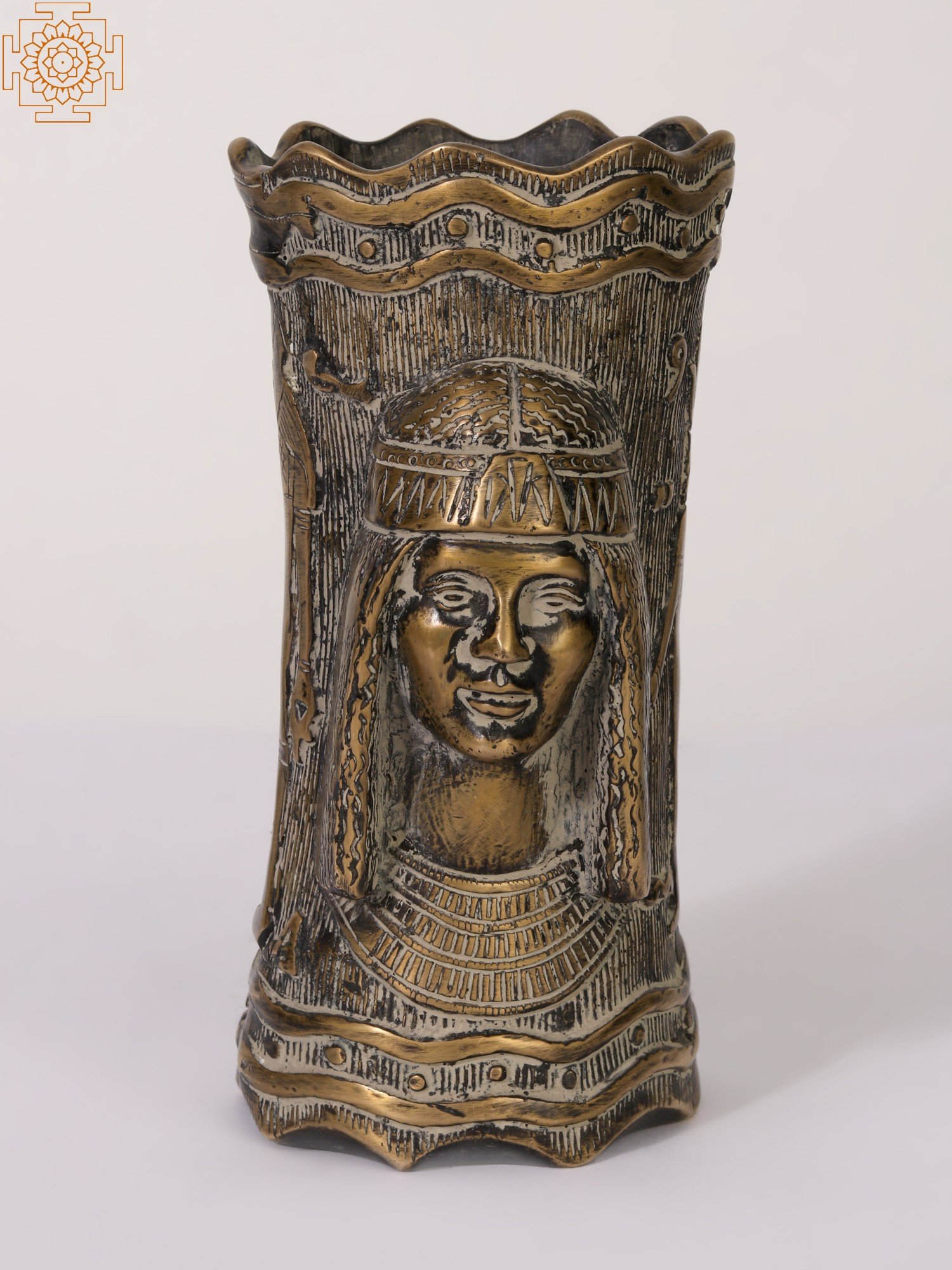The image features an ancient-looking bronze artifact, resting against a pure white backdrop. The object appears to be a vase-like statue with a distinct patina, indicating its age. At the top, it has an opening with wavy edges, and running vertically down the sides are ridges that create a textured surface. In the center of the artifact, a detailed 3D face is prominently displayed. The face, possibly female, wears a headband and a necklace reminiscent of ancient Egyptian adornments. Black or white lines, likely signs of aging, trace down the vertical ridges of the vase. In the top left corner of the image, a symbol is visible, featuring a round floral or star design enclosed within a box-like pattern. This intricate symbol adds to the artifact's air of ancient royalty and cultural significance.